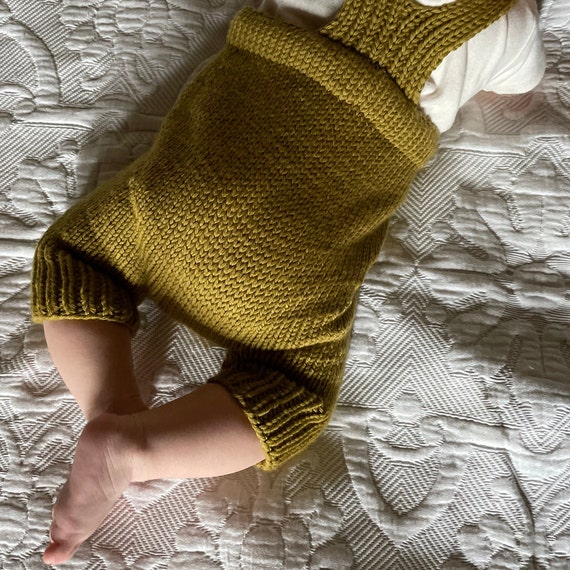The image depicts a baby lying on its stomach. The view is from the shoulders down, showing the baby’s back and legs. The baby is dressed in a white onesie and a knitted pinafore made of thick yarn, appearing brown or dark olive green in color. The pinafore only extends to the knees, leaving the lower legs exposed, which are crossed at the ankles, with the right leg over the left. The baby is positioned diagonally on a blanket that is predominantly white and grey, featuring embroidered floral patterns and striped background accents.